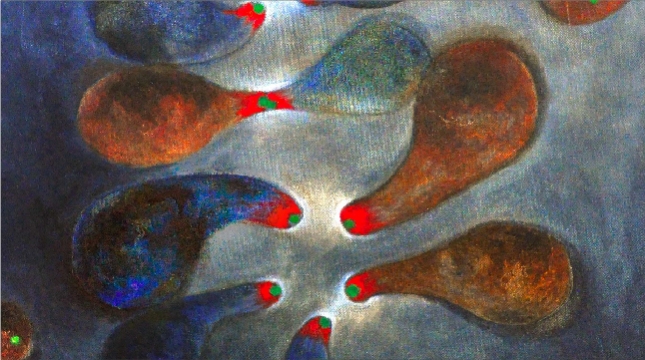This rectangular canvas painting, measuring about four to five inches wide by three inches high, features a vividly detailed scene. The background transitions from deep navy blue and dark grays on the left to lighter blues and grays on the right, rendering a gradient effect that enhances the depth of the artwork. Horizontal and crisscross lines of the canvas are faintly visible across the entire piece.

Prominently displayed are several gourd-shaped figures scattered throughout the painting. These shapes, resembling either squash or pears, have round bulbous bodies tapering into thin necks, all adorned with red tips and green dots at the ends. On the left side, the composition includes a sequence of gourds: a blue one above, an orange one in the center, and two more blue gourds at the bottom. These leftward-facing forms are accented with white highlights behind them. 

On the right side, similar shapes appear, with two orange gourds below a blue gourd, also facing left. One of the blue gourds on the left connects with a lighter blue and green gourd on the right, forming a visual link where their green-tipped ends meet. Additional floating gourds of varying shades add to the painting's dynamic balance and texture, exhibiting meticulous shading and intricate detailing. The overall aesthetic suggests a careful blend of color and form, creating a captivating visual experience.